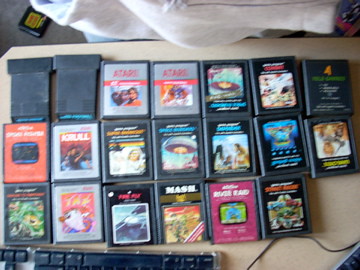The image features a small table adorned with various items related to gaming. At the center of the table, several red cartridges catch the eye, each displaying vibrant, retro-style designs. Scattered around the cartridges are an assortment of game purchase receipts, adding a sense of recent activity and excitement. The background reveals a card screen, possibly showing game details or settings, further enhancing the scene's gaming ambiance.